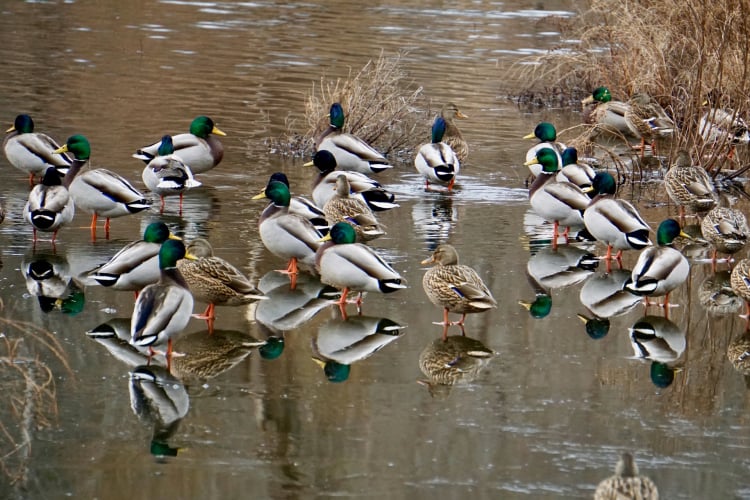This wildlife photograph captures a serene autumn or winter scene at a pond, where approximately twenty mallard ducks are gathered in the shallow, reflective water. The stillness of the pond accentuates the mirror image of the ducks, creating a captivating symmetry with the ripples gently distorting their reflections. The male mallards, with their gleaming green or bluish-green heads and grey bodies adorned with brown lines, dominate the scene, while the brown-feathered females are interspersed among them. A couple of ducks display distinctive blue heads, adding variety to the assembly. The background features the subtle presence of brown, dried-back vegetation along the edges of the pond, enhancing the seasonal atmosphere.